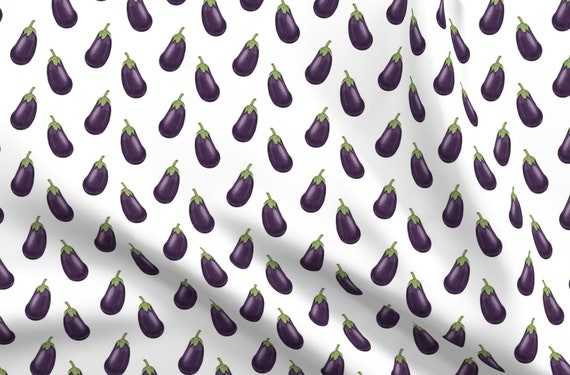The image captures a piece of white fabric that is adorned with a uniform, latticed pattern of eggplants. Each eggplant is artistically drawn, bearing a purple body and a green stem that consistently points upward. The eggplants are arranged in vertical lines, with each line alternating the orientation of the eggplants diagonally left and right, creating a mirrored effect. This pattern is evenly spaced, with no eggplants touching each other, and offset vertically by half, forming a distinctive lattice. The fabric itself has visible folds in the lower right and along the bottom edge, casting small shadows that confirm its soft, flexible nature. The overall impression is reminiscent of an intricately designed wallpaper or wrapping paper, dotted with what seems to be hundreds of these small, jelly bean-sized eggplants.